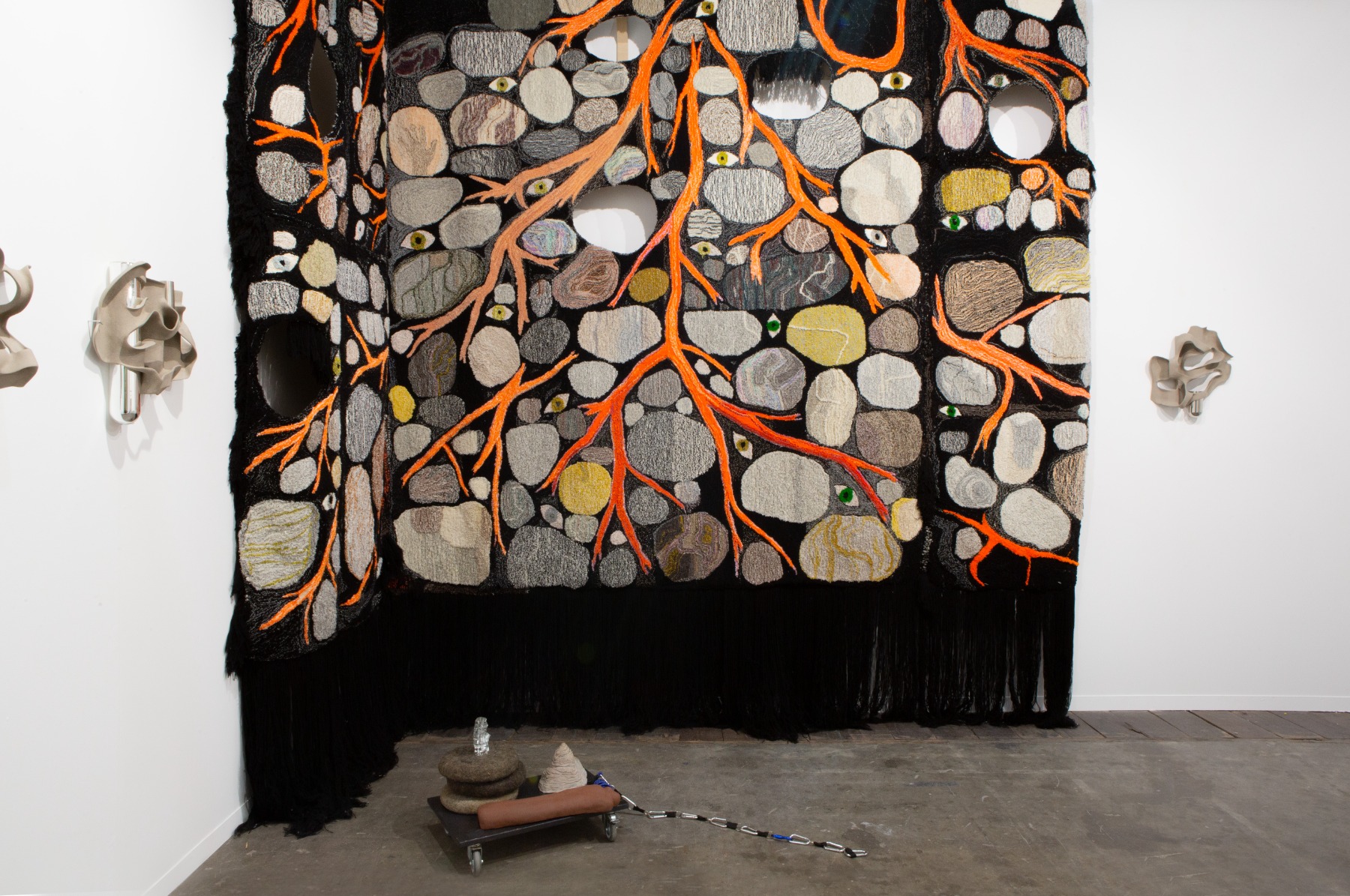This color photograph captures a captivating corner of a contemporary art exhibit set in a museum. The room features white walls and a gray concrete floor, lending a minimalist backdrop to the intricate artwork. Dominating the scene is a monumental black fabric installation that extends from the ceiling, cascading along one wall and partially down an adjoining one, pooling slightly on the floor with strands of black fringe at its base. 

Affixed to the black backdrop are an array of meticulously detailed pebble shapes in naturalistic hues such as grays, whites, and yellows, some marbled with veins. Interwoven among these stones are vibrant orange and reddish roots, reminiscent of tree or plant roots, which elegantly thread through the composition. Adding a surreal element, eye shapes peek out from the pebbles, resembling protective evil eyes.

In front of this textile art, on the floor, sits a low, wheeled cart adorned with actual stones, a leather piece, and an oval orange object, connected by a blue and white rope. Additionally, the white walls are accented by three small, tan, abstract sculptures resembling mask forms, enhancing the exhibit's depth and intrigue. This elaborate arrangement beautifully merges natural elements with crafted artistry, creating a visually rich, immersive experience.